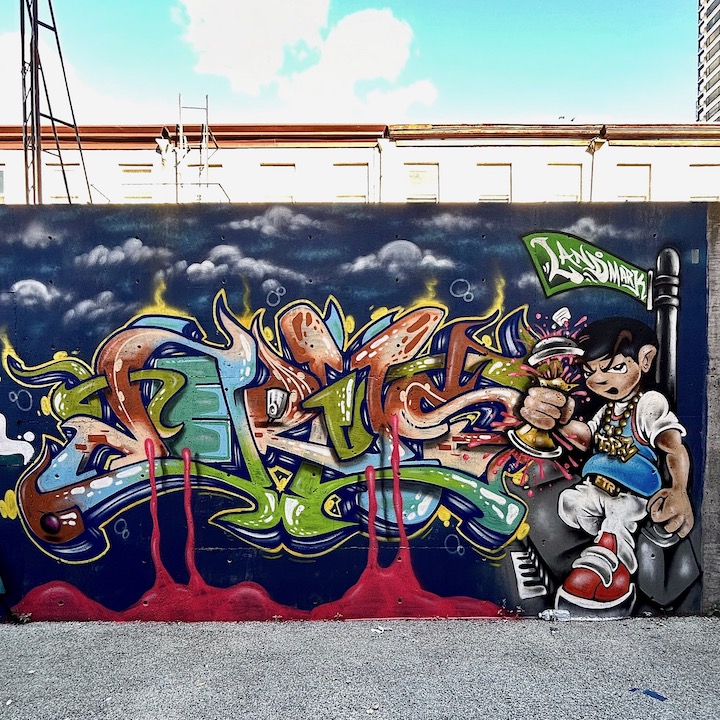The image captures a vibrant piece of graffiti painted on an outdoor wall, seemingly on a sunny day. The centerpiece of the mural features a cartoonish African American boy with short dark hair, depicted with an intense, menacing expression, emphasized by arched eyebrows. On the left side, he wears a white short-sleeve t-shirt topped with a blue basketball jersey and a gold medallion necklace inscribed with the word "Torts." His outfit is completed by a belt with the letters "FTR," white pants, and big red basketball shoes. 

The boy's right hand visibly squeezes a can, from which pink liquid explosively spurts out, signifying his firm grip. Above him, a street sign reads "Landmark," adding an urban element to the artwork. The graffiti's text, stretching from left to right, is indistinct and rendered in multiple colors, including brown, green, and blue. The mural's background features a dark blue sky filled with grayish-white clouds, while the bottom of the image shows a drawing of red liquid or goo. This intricate, colorful display stands out against the city backdrop, making it a striking example of traditional graffiti art.